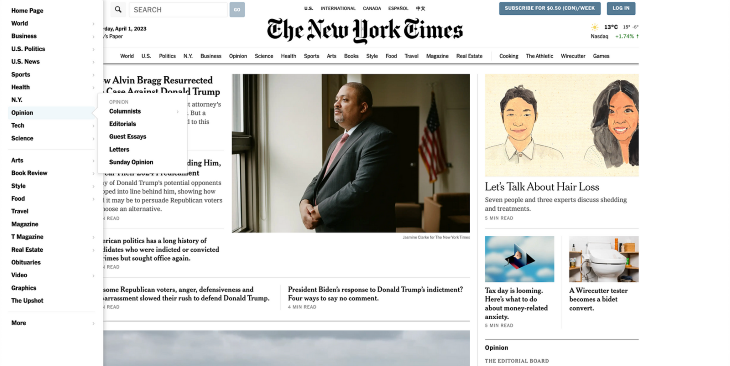The image showcases the New York Times website. On the left side of the page, there is a vertical menu that lists various sections of the site: Homepage, World, Business, U.S. Politics, U.S. News, Sports, Math, Health, NY, Opinion, Tech, Science, Arts, Book Review, Style, Food, Travel, Magazine, Real Estate, Obituaries, Video, Graphics, The Upshot, and Mars. The selected section is "Opinion," highlighted prominently.

At the top of the page, the recognizable New York Times logo is displayed in its signature font. Below it, within the Opinion section, there is a pop-out sub-menu featuring the categories: Opinion, Columnists, Editorials, Guest Essays, Letters, and Sunday Opinion. This menu partially obscures an article displayed in the center of the page.

The visible portion of the article includes a picture of Alvin Bragg with a headline that appears to discuss Alvin Bragg resurrecting a case against Donald Trump. However, the full article title is obscured by the pop-out menu. Additionally, there is another article headline visible, reading, "President Biden's response to Donald Trump's indictment: Four ways to say no comment."

On the right side of the page, there is a sidebar with content that might include various headlines or articles; one mention stands out - "Let's talk about hair loss."